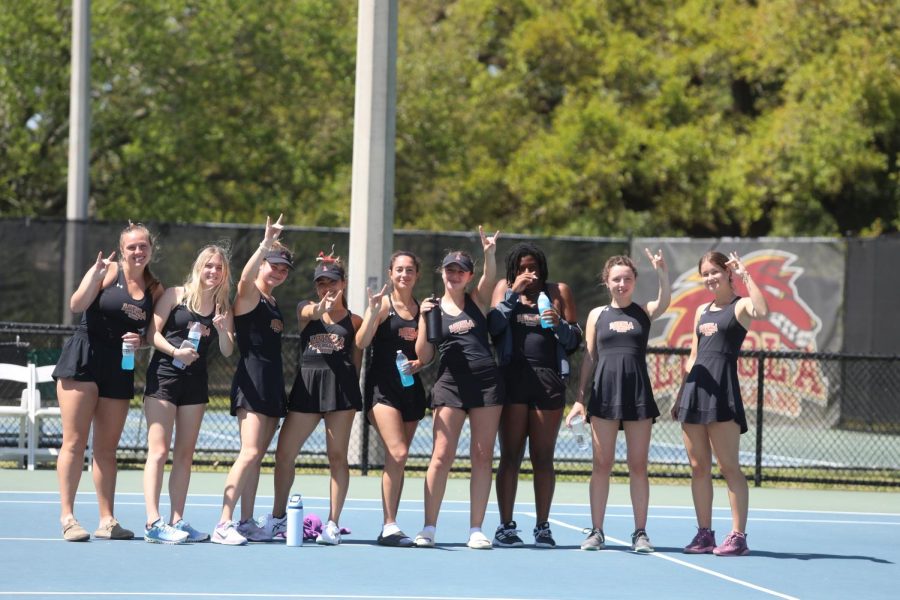This horizontally aligned rectangular image captures a lineup of nine or ten teenage girls standing on a blue tennis court, distinguished by white stripes. They appear to be part of a tennis team, wearing black athletic uniforms, which include varying combinations of tennis skirts, shorts, and tank tops. Some of the girls are adorned with ball caps or visors, while others are not. Each girl is making a peace sign with her hand. Most of them are holding blue-labeled Gatorade bottles, and some white water bottles with pink items scattered on the ground. All but one girl, who wears black shoes, are sporting white shoes, and one girl on the far end wears pink and black shoes. A black girl in the lineup stands out with black shoes, and a girl next to her is seen in black slides. 

In the background, the blue court is enclosed by a black chain-link fence. Beyond this fence, there is another tennis court and patches of green grass. Covering another section of fencing is a black material featuring a logo that includes the letters "L-O-L-A" and depicts a red wolf or horse, emphasized with yellow and white outlines. The scene is further framed by tall green trees with visible brown branches, providing a lush backdrop.